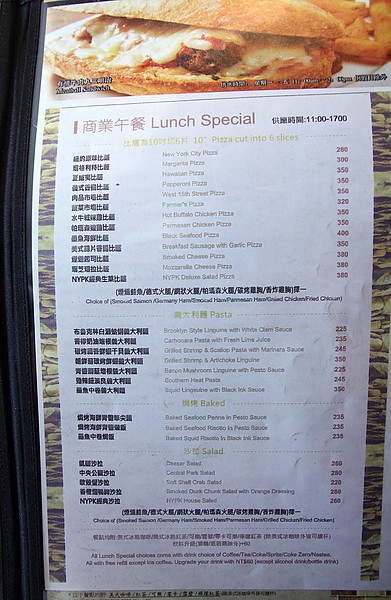A vibrant, color photograph showcasing a detailed menu in portrait orientation. The menu itself is richly adorned, featuring a sleek black border that frames the content within. At the top of the menu, a narrow, eye-catching cropped photograph highlights a delectable sandwich. The sandwich, crafted from an oblong bun, is generously filled with succulent meatballs or another form of meat, drenched in a savory red sauce and topped with melty, white cheese. 

Beneath this appetizing image lies a prominent white panel headlined with the words "Lunch Special." The menu text is bilingual, presented both in English and an Asian script, catering to a diverse clientele. 

The menu is systematically organized into various sections: "Pizza," "Pasta," "Baked," and "Salads." Each item is meticulously listed with the Asian script on the left, the English translation prominently centered, and the prices, assumedly, displayed in striking red numerals on the right. This detailed layout offers a clear and appetizing preview of the culinary delights available.